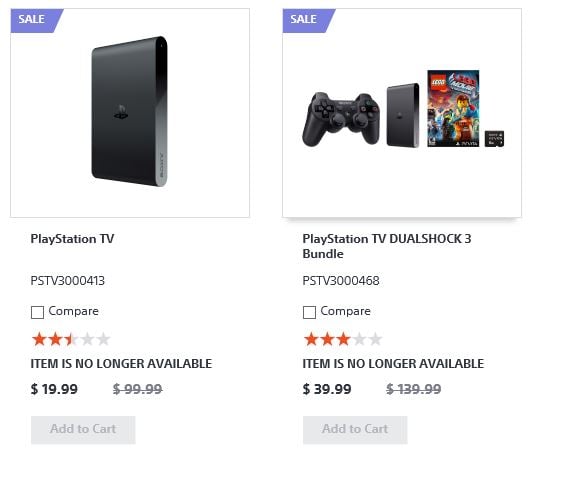This image features a screenshot comprising two distinct sections related to PlayStation products. On the left side, there's a display of the standalone PlayStation TV unit, marked with the serial code PSTV 300413. This product, originally priced at $99.99, is on sale for $19.99. Despite its discounted price, the "add to cart" option is inactive, and the item is indicated as no longer available. The product garnered a rating of 2.5 out of 5 stars. 

On the right side, the screenshot presents the PlayStation TV DualShock 3 bundle, identified by the serial code PSTV 300468. This bundle, which includes a DualShock 3 controller and a video game, was originally priced at $139.99 and is on sale for $39.99. Like the standalone unit, the "add to cart" option for this bundle is also grayed out, and the item is marked as no longer available. This bundle has a slightly higher rating, with 3 out of 5 stars.